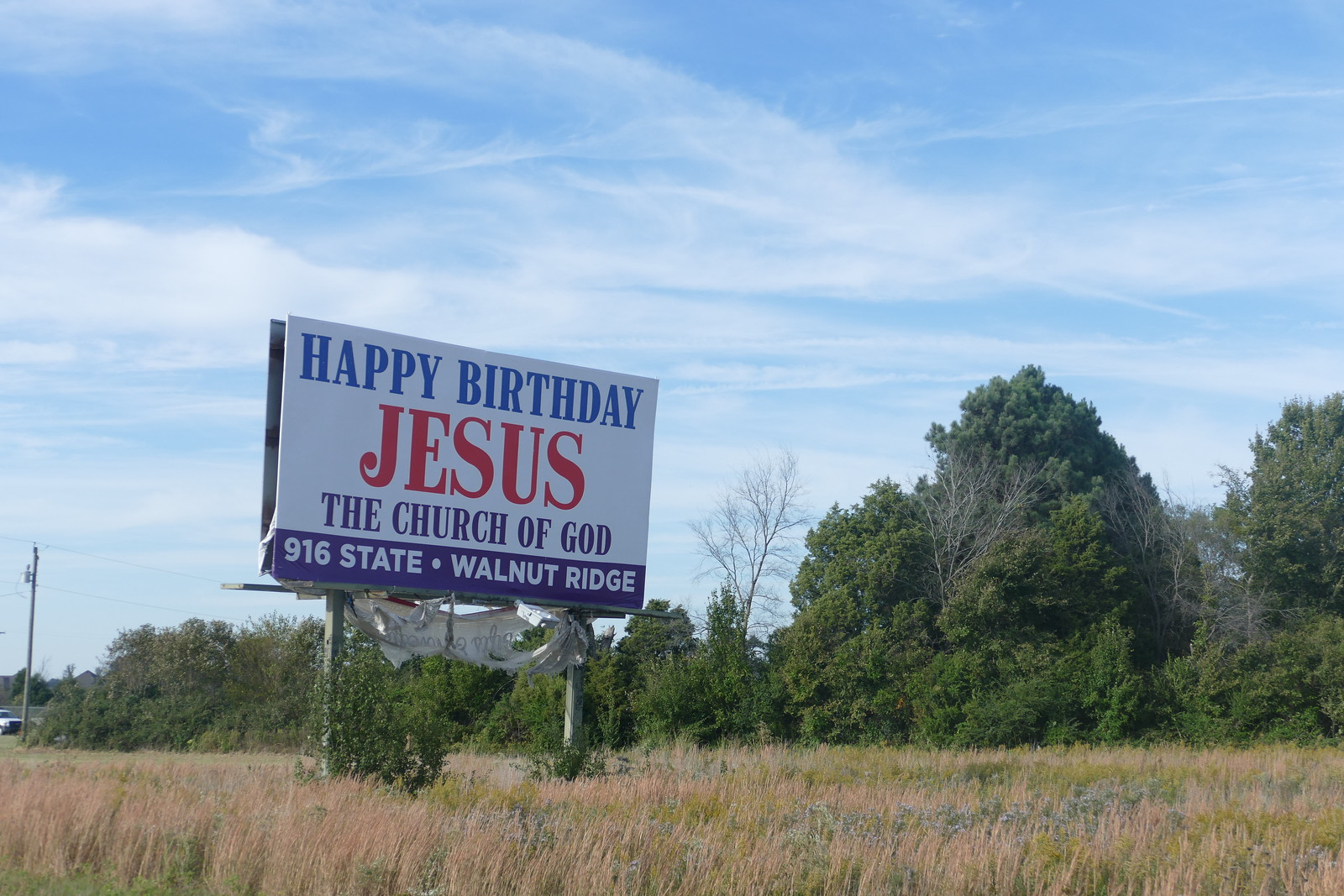A serene blue sky dotted with wisps of white clouds stretches over a picturesque landscape. In the background, a dense arrangement of lush green trees interspersed with dormant, branchy ones creates a vibrant and textural panorama. To the far left of the scene, a power line pole extends upward, with lines crisscrossing the sky. Below, various cars add a sense of everyday life to the tranquil setting. The ground in the foreground presents a mosaic of dry and green grass.

Prominently featured in the center is a large sign framed by greenery. The sign reads: "Happy Birthday Jesus, The Church of God, 916 State, Walnut Ridge," with text arranged in white against a backdrop that transitions from blue at the top, red in the middle, and blue again toward the base. The festive message is complemented by the legs of a person visible on either side of the sign, adding a human touch to the composition. Beneath the sign, a tattered banner flutters, hinting at the passage of time and the elements.